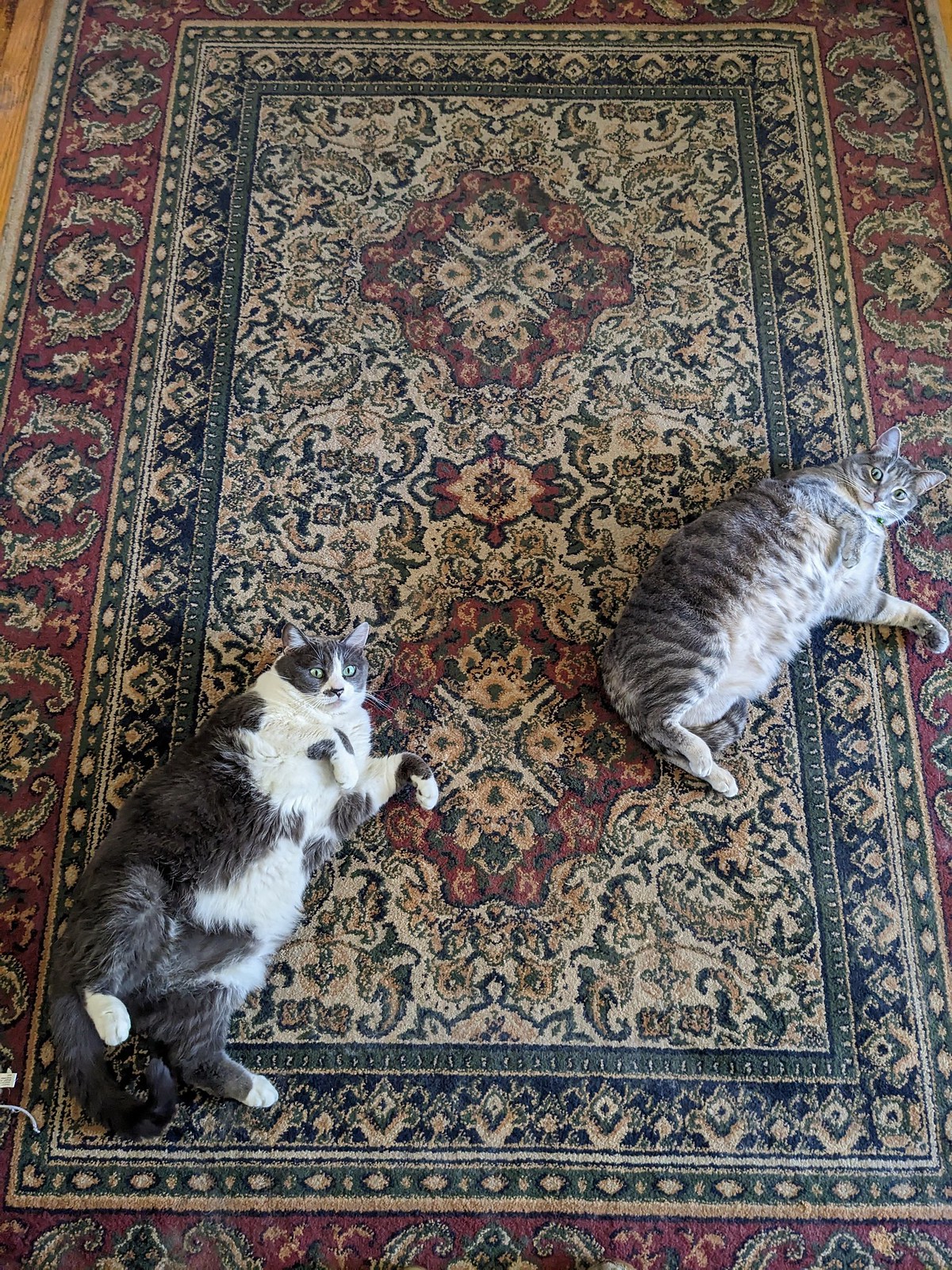This photograph showcases two cats lounging on an elaborate Persian rug that features a rich tapestry of colors and intricate patterns. The rug, evoking an old-world charm, is well-worn, possibly from the cats' frequent use. Dominated by a red outer layer, a thin green layer, a blue section, and a large yellow layer adorned with floral and geometric designs, the meticulously detailed rug forms a striking backdrop. The image is shot nearly vertically, capturing both cats lying on their sides within the lower half of the frame. Positioned on the left, one cat flaunts a distinctive gray and white coat with a gray face mask, white belly, and white paws. To the upper right, a gray and black striped cat lies partially reclined. Both cats extend their front paws slightly and gaze directly at the camera, possibly napping or playfully posing on the wooden floor beneath the rug. The serene and captivating moment highlights the cats' relaxed demeanor on this luxurious, vividly designed rug, with no other objects visible in the frame.